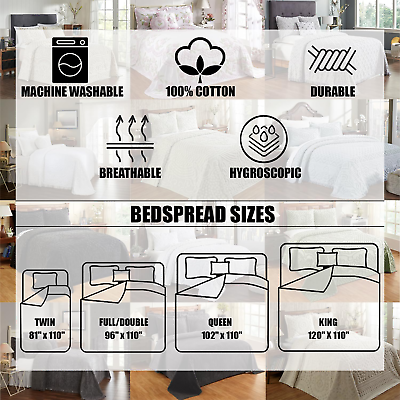The image features a white, semi-transparent pamphlet overlaid on a background of twelve different photos of beds, arranged in a grid of three rows. Each bed displays various bedspreads, showcasing different colors and flooring types. The pamphlet is detailed with icons and text that describe specific qualities of the bedspreads. From left to right, the top half lists features such as "Machine Washable" with an icon of a washing machine, "100% Cotton," "Durable," "Breathable," and "Hygroscopic," all in black and white. Below this, the middle section of the pamphlet details bedspread sizes according to different bed dimensions: Twin (81x110), Full/Double (96x110), Queen (102x110), and King (120x110). The design serves to combine practical information about bedspread features and sizes with illustrative imagery of how they look in various bedroom settings.